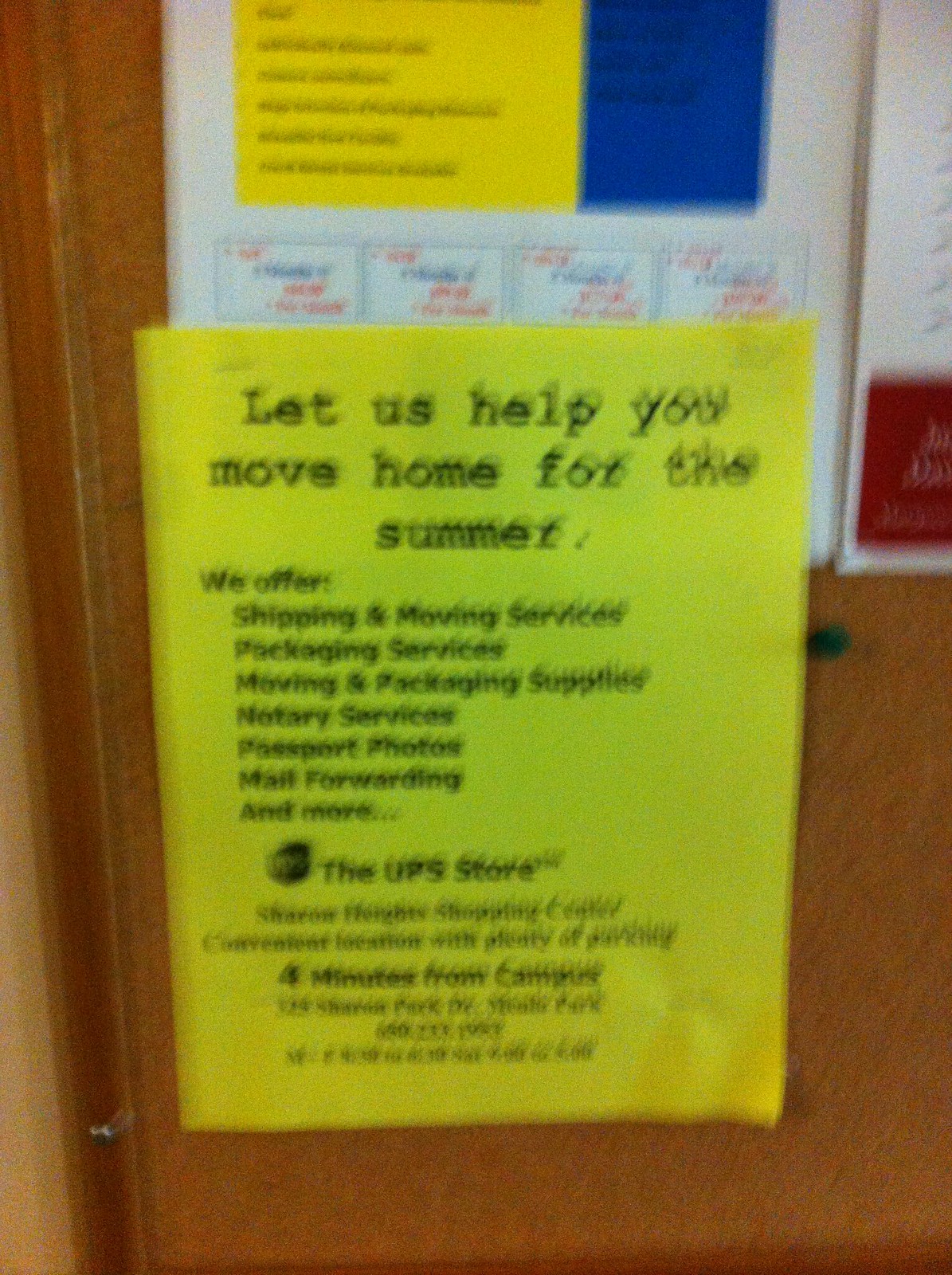The image captures a real-life notice board, characterized by its blurry and grainy quality. Dominating the board is a prominently positioned yellow notice from The UPS Store, featuring the UPS logo to its left. The main text reads, "Let us help you move home for the summer," followed by bullet points highlighting their services, including shipping and moving services, packaging services, moving and packaging supplies, notary services, passport photos, mail forwarding, and more. However, due to the image's blurriness, the additional 6-7 lines of text are illegible. Behind this notice is another paper with a yellow and blue column and four indistinguishable options listed. The board also features the partial left edge of another paper and is held together with a lone thumbtack, though the papers appear to be primarily stapled to the brown corkboard. Surrounding the board is a dark brown frame, and barely visible to the side is the beige wall of the room.